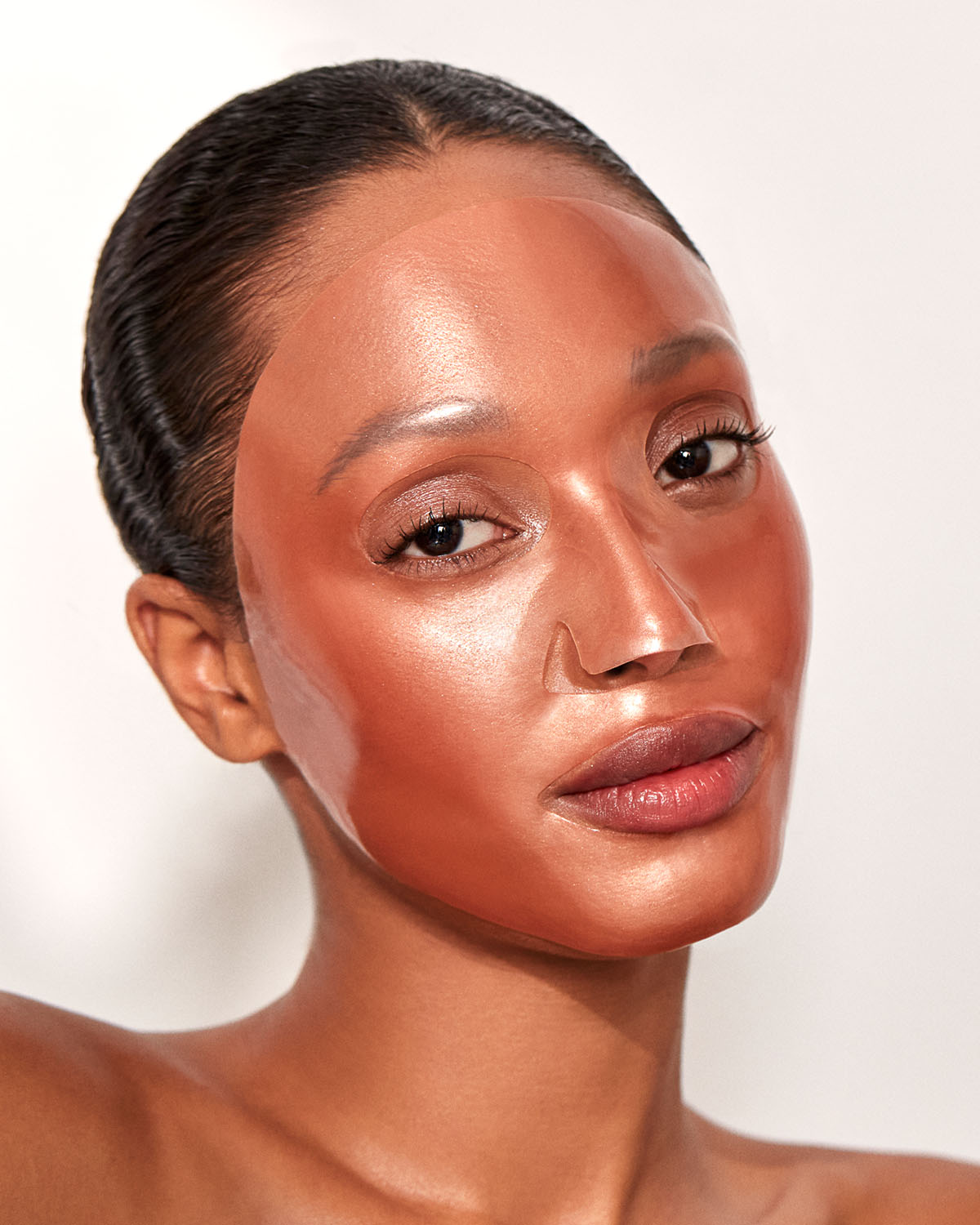This is a close-up image of a light brown-skinned Black woman with short, neatly parted dark brown hair pulled back and slicked above her ears. She is wearing an oval-shaped, transparent plastic face mask that covers almost her entire face except for an opening beneath her nose, allowing her nostrils to be visible. The mask contours over her cheeks, forehead, nose, and around her eyes, extending to her left ear without covering it. The mask creates an illusion of changing her nose's appearance. The woman has dark oval-shaped eyes highlighted with light eyeliner and long lashes, and her lips are full and dark red-pinkish. Her head is slightly tilted, but she is looking directly at the camera with a very slight, closed-mouth smile. She is shown from the shoulders up, and the bare tops of her shoulders are visible against a white background, with no clothing apparent in the frame.